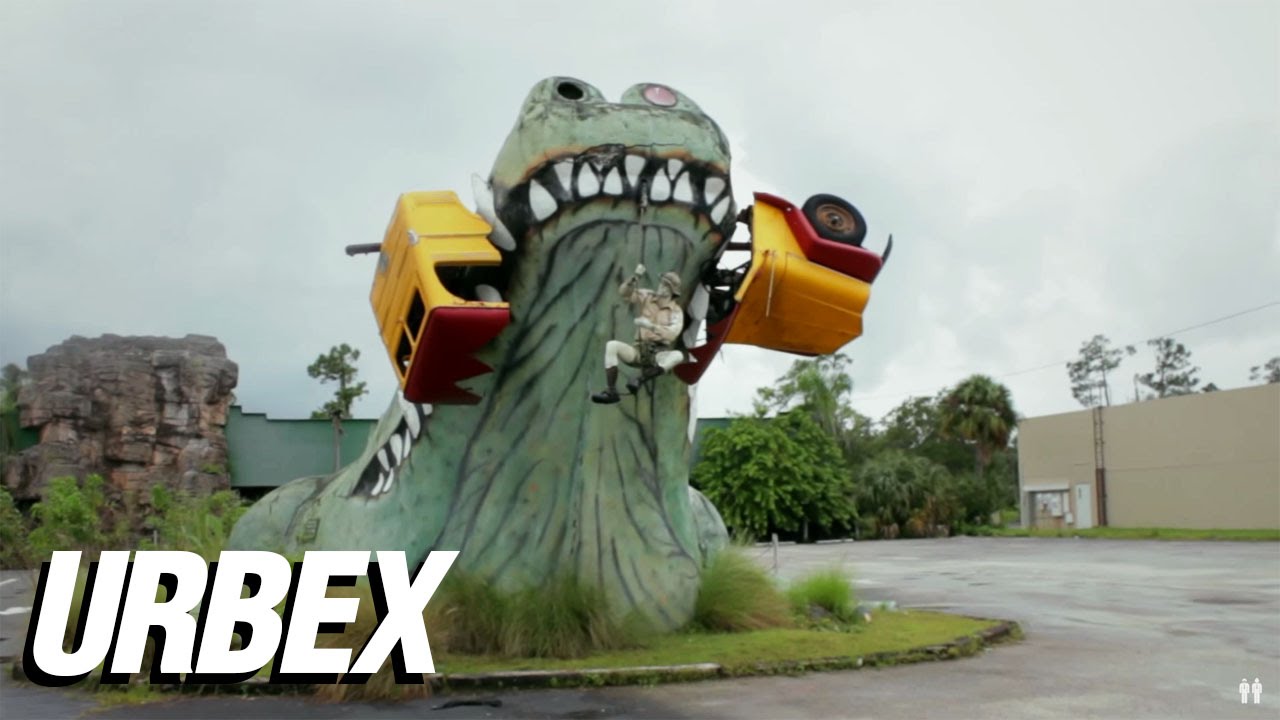The image depicts an overcast day at what appears to be an abandoned amusement park, characterized by its weathered and desolate appearance. Dominating the scene is an enormous, dramatic sculpture of a green alligator head with black accents, its wide-open mouth revealing sharp white teeth. The alligator is gripping a school bus—painted black, yellow, and maroon—in its mouth, seemingly crunching it in two. 

Central to the image, there's an individual, outfitted in black boots, white pants, a cargo vest, shirt, and hat, hanging from a rope; further inspection reveals this figure to be a statue styled like an adventurer, reminiscent of Indiana Jones. Surrounding this central attraction, there's a gray asphalt area, possibly a parking lot or street, with a circle of green grass and patches of leaves.

The setting is framed by a variety of background details: a sand-colored building to the right, segments of a weathered stone wall, a green elevated bridge, and electric wires. Nearby, bushes, trees, and a mountain wall add to the scene's rugged ambiance. In the lower left corner, the word "URBEX" is prominently displayed in large white block letters against a black background, while in the lower right corner, a watermark features two white pedestrian figures. The overall scene evokes a sense of exploration and decay, typical of urban exploration (urbex) photography themes.